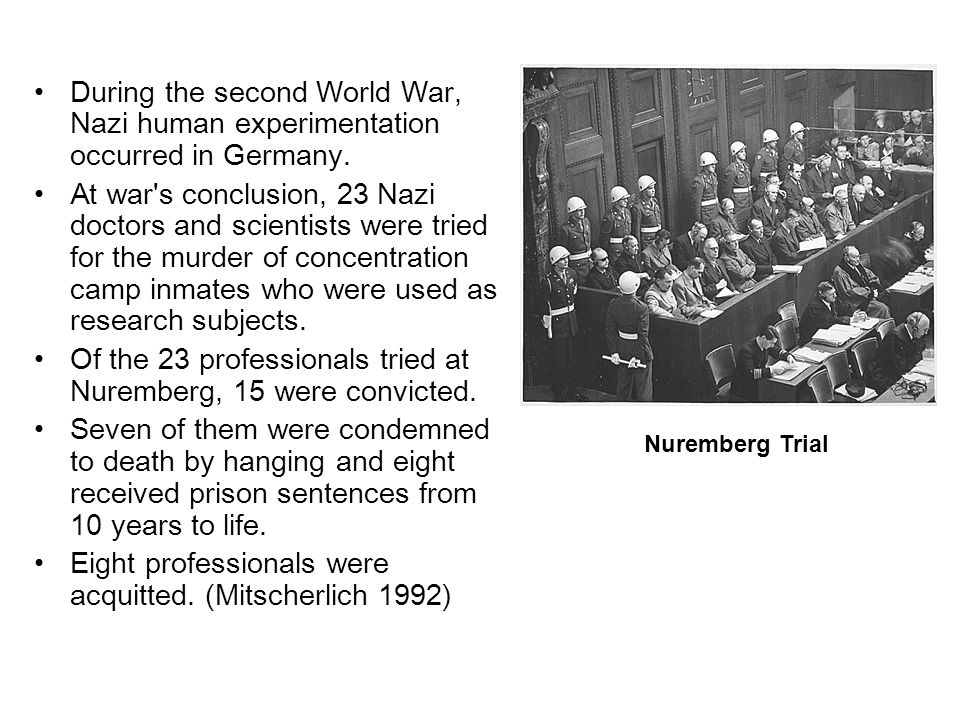This image appears to be a black-and-white slide from an educational presentation or an online article, focusing on Nazi Germany and the Nuremberg Trials. The left side of the image presents five bullet points in black sans-serif font, on a plain white background. The bullet points detail the following: 

1. During the Second World War, Nazi human experimentation occurred in Germany.
2. At the war's conclusion, 23 Nazi doctors and scientists were tried for the murder of concentration camp inmates who were used as research subjects.
3. Of the 23 professionals tried at Nuremberg, 15 were convicted.
4. Seven of them were condemned to death by hanging, and eight received prison sentences ranging from 10 years to life.
5. Eight professionals were acquitted.

The citation "(Mischerlich, 1992)" follows these points. 

On the right side, there is a black-and-white photograph from the Nuremberg Trials. The photo, set in a courtroom, shows military personnel wearing helmets and armed with guns. Visible behind them is wood paneling and a group of individuals possibly comprising the jury, counsel, or other trial participants. The image emphasizes the solemnity and formality of the historic proceedings.